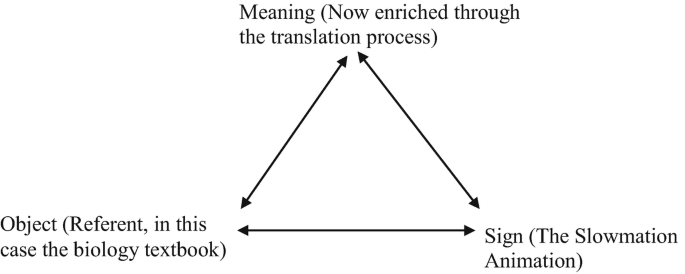This black and white diagram features three lines forming a triangle, each line adorned with arrows at both ends. At the top of the triangle is the word "MEANING" in black lettering, accompanied by the phrase "(now enriched through the translation process)" in parentheses. The bottom left corner is labeled "OBJECT" with the detail "(referent, in this case the biology textbook)" in parentheses. The bottom right corner reads "SIGN" with the explanatory note "(the slow motion animation)" in parentheses. The lines of the triangle include a horizontal base and two diagonal lines connecting the base to the apex, all set against a white background. This simple yet informative graph-like figure visually represents the relationship between meaning, object, and sign.